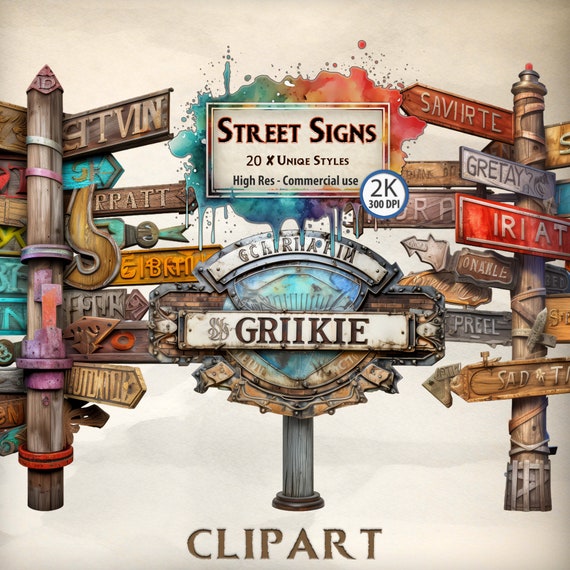This is a detailed graphic illustration of assorted street signs presented as clip art. The image features three wooden signposts adorned with a multitude of street signs, except for the center post which bears only one sign. Each sign displays various text, some in English and others resembling foreign words or nonsensical text like "gratae," "greeky," "SAVIRTE," and "GRITE," alongside typical street sign shapes such as arrows. At the top, in a bold off-white rectangle with black text, it reads "Street Signs," followed by "20X UNIQUE STYLES, HIGH-RES, COMMERCIAL USE." Adjacent to this text box, a white circle with a blue border indicates the quality, stating "2K, 300 DPI." The background of the illustration is a muted gray or beige color, providing a neutral canvas that highlights the colorful and varied street signs. At the bottom of the image, brown lettering spells out "clip art," emphasizing the graphic nature of the illustration.